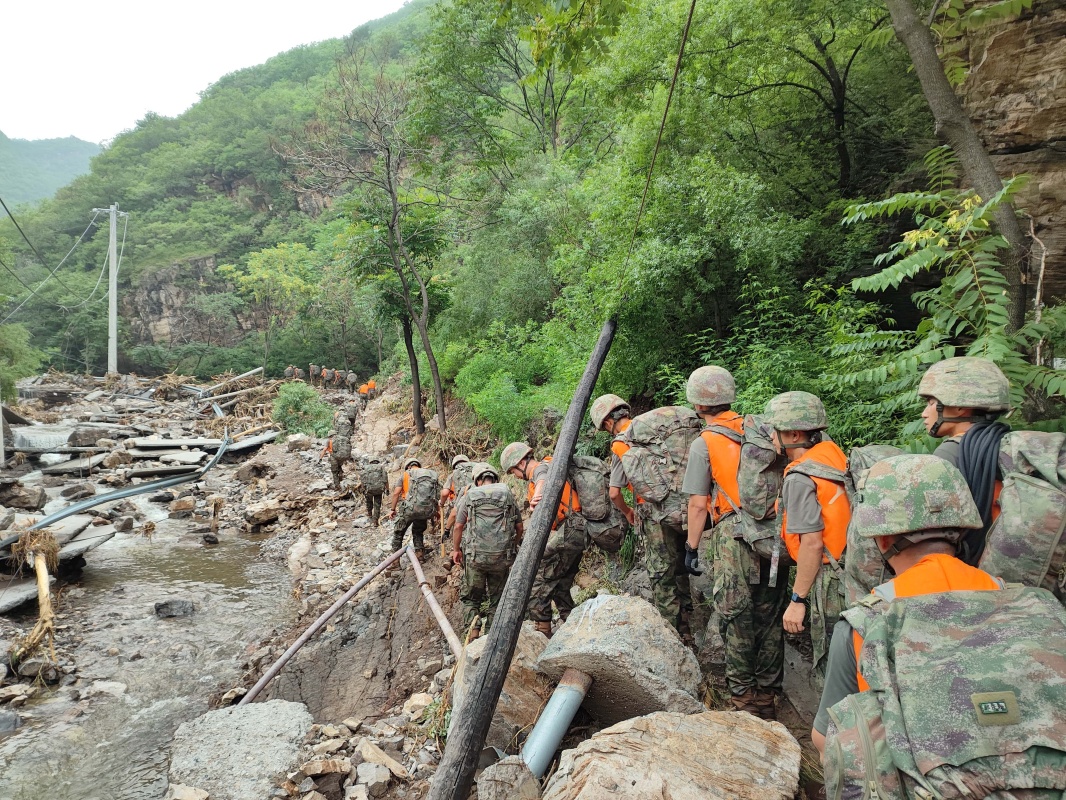In this outdoor scene, the upper left corner of the image reveals a white sky above a hill covered in greenery. The left side of the image looks muddy, reminiscent of the bottom of a drained river, and is dotted with broken chunks of concrete, one of which is turned upside down with a metal pipe protruding from it. On the right side, a rock cliff looms over the scene, with a group of soldiers clad in camouflage uniforms, orange safety vests, and camo helmets. They are walking from the lower right towards the center, forming a long line along the muddy, rocky edge of the cliff, which is adjacent to a stream of water. Scattered power lines and a droopy power pole indicate the aftermath of a natural disaster. The soldiers appear to be navigating the debris-strewn landscape, suggesting they are involved in a rescue or recovery operation amidst the damaged, gray and brown terrain.